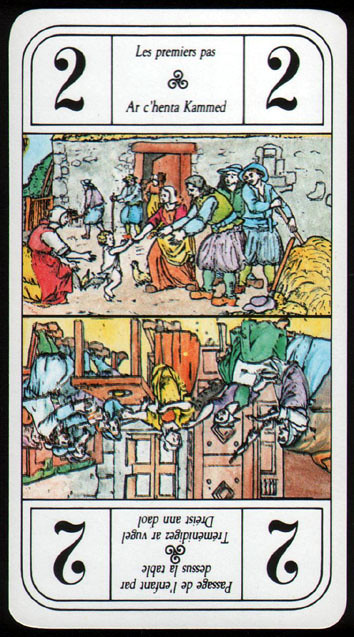**Detailed Caption:**

This intriguing card appears quite unusual, presenting prominent numerical values. It showcases the number "2" at all four corners, with the two at the top left and right appearing normally, while the bottom two numbers are displayed upside down. The card itself is split into two distinct halves, each bearing a different image which requires inversion to view correctly.

The top half of the card illustrates a scenic depiction involving a group of people gesturing towards a young boy. Behind them stands a house, adding depth to the setting. When inverted, the bottom half reveals an interior scene where a woman appears to be serving several men. In the background, several women are present, one of whom, possibly a nun, exhibits an angry gesture towards the serving woman.

The card features French text interwoven with the images. At the top, it reads, “Les premiers pas l'argente comed.” Along the dividing line between the images, it says, "Passage de l'enfant par dessus la table. Tremendis albrogol dresse en dalle."

This card, distinguished by its divided imagery and dual perspectives, as well as the presence of text, conveys both visual and linguistic narratives that invite closer inspection and interpretation.